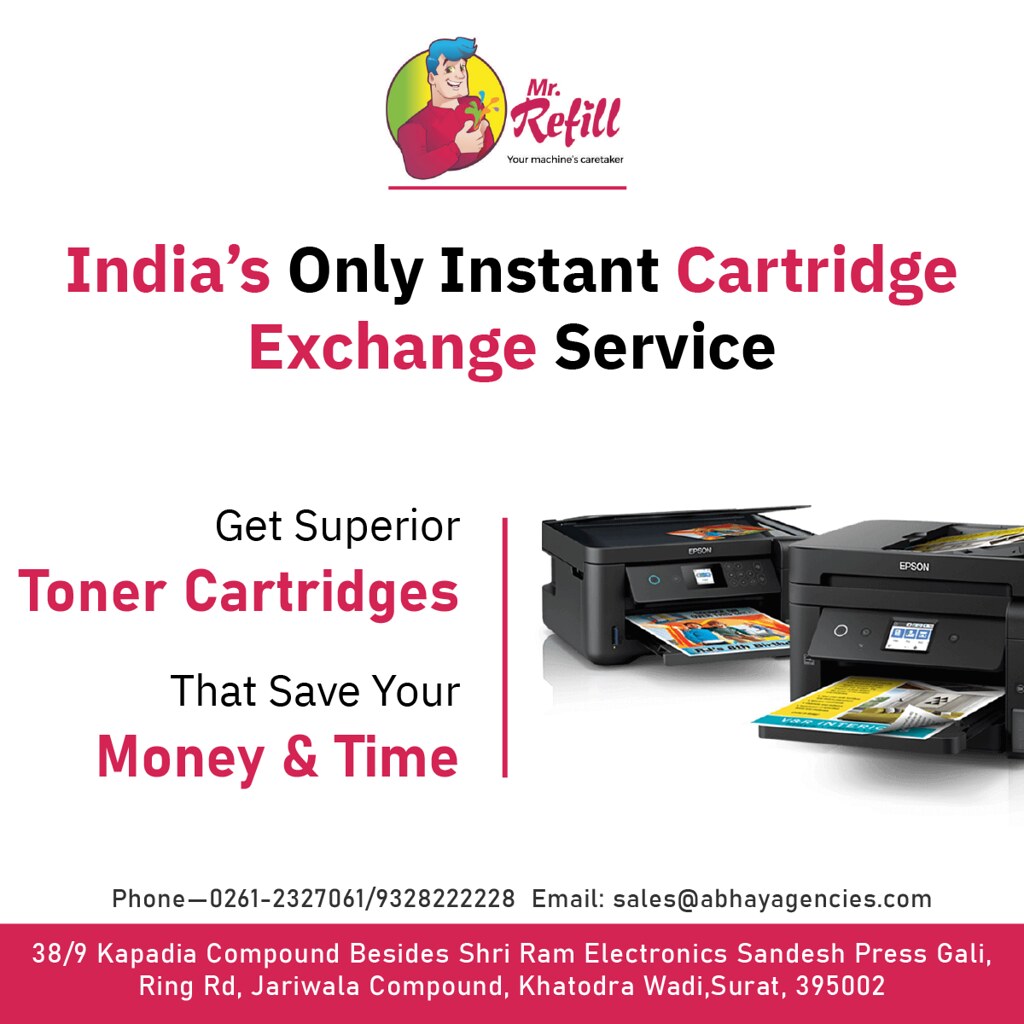This is an advertisement poster for Mr. Refill, India's only instant cartridge exchange service. Dominating the top center is the company mascot, a cartoon man with blue hair, wearing a red long-sleeve shirt. He has his thumb and index finger close together, emitting colorful streaks of green, blue, orange, red, and purple. The company's name, "Mr. Refill," is displayed in red font with a heart dotting the 'i', followed by the tagline "your machine's caretaker" in black text with a red underline. Below that, the text reads "India's only instant cartridge exchange service." On the right side of the poster, two black Epson printers are visible, filled with vivid and colorful printed sheets in their trays, with LED lights lit up indicating they are at work. The left side features the text "get superior toner cartridges" in black and red, along with "that save your money and time" in black. At the bottom of the poster, there is contact information including a phone number, email address, and physical address, all against a white background with black and red text.